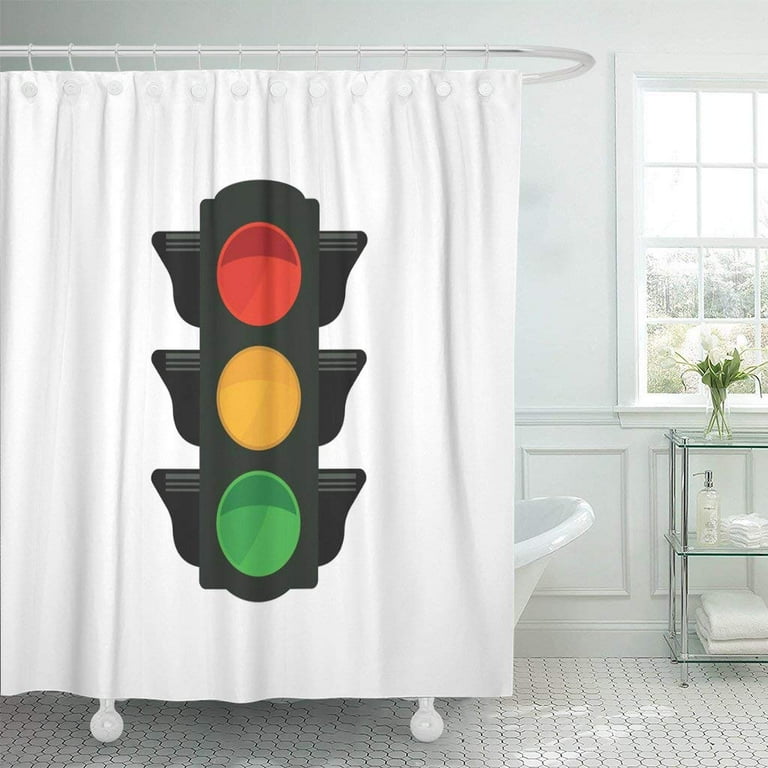The bathroom features a predominantly white color scheme with touches of green, primarily from a plant. Dominating the scene is a large white bathtub with claw feet, encircled by a white shower curtain. The shower curtain is adorned with a vivid, large traffic light graphic, showing a red light at the top, a yellow light in the middle, and a green light at the bottom on a black background. Suspended by an oval chrome rod near the ceiling, the shower curtain adds a playful element to the space.

To the right of the bathtub, there's a window without curtains, revealing a sunny day with hints of greenery outside. Below the window stands a chrome, three-tiered glass shelf. The top shelf holds a vase with white flowers and green leaves, the middle shelf contains what appears to be a lotion bottle and some other white items, while the bottom shelf has two neatly folded white towels.

The bathroom floor features small decorative ceramic tiles, contributing to the clean, bright ambiance of the room. Despite minor differences in the descriptions of the weather outside, the scene conveyed is of a well-lit, white-accented bathroom with a touch of greenery and whimsical decor.